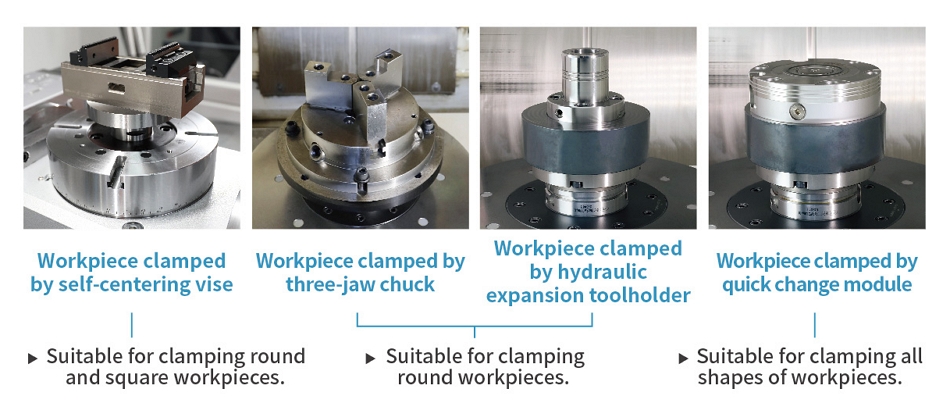The image displays detailed instructions about different clamping techniques used in machinery, depicted through four left-to-right sequential photographs. Each image has blue and black writing beneath them, specifying the type of workpiece holder and its suitability. 

- **First Image:** A shiny metal circle with bolts and metal pieces extending outwards, labeled "Workpiece clamped by self-centering vise," suitable for clamping both round and square workpieces.
- **Second Image:** A similar metal circle, described as "Workpiece clamped by three-jaw chuck," suitable for clamping round workpieces.
- **Third Image:** Another metal circle, dark gray in color with a bolt, marked "Workpiece clamped by hydraulic expansion tool holder," also suitable for clamping round workpieces.
- **Fourth Image:** A large silver metal cylinder with dark gray metal around it, identified as "Workpiece clamped by quick change module," suitable for clamping all shapes of workpieces. 

All metal pieces look new and are presumably intended to illustrate the practical application of these clamping tools for potential buyers.